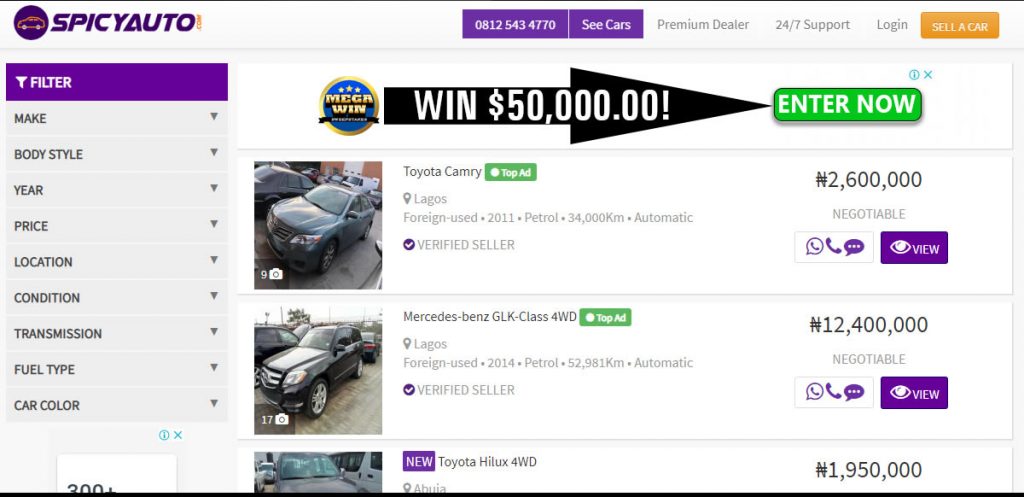This image depicts a web page from Spicy Auto, a site dedicated to automobile sales and services. In the upper left corner of the screen, the brand name "Spicy Auto" is prominently displayed in bold purple text, accompanied by a simplistic round avatar depicting a side-view drawing of an automobile. 

To the right of the brand name, there are two adjacent buttons in the same purple hue. The first button features a phone number in white text: "08-12-543-4770," while the second button is labeled "See Cars." Continuing to the right, written in gray text, are the words "Premium Dealer," "24-7 Support," and "Log In." At the far right of this top section, there is an orange button with white text reading, "Sell a Car."

Below the brand's logo and name, on the far left, is a short, purple banner labeled "Filter" in white text. This banner precedes a vertical list of filter options: Make, Body Style, Year, Price, Location, Condition, Transmission, Fuel Type, and Car Color.

To the right of these filters, there is a vertical list featuring different vehicles for sale, such as a Toyota Camry, a Mercedes-Benz GLK Class 4-wheel drive, and a Toyota Hilux 4-wheel drive. Each vehicle listing includes pricing information as well as options to call, text, or view further details.

Above the vehicle listings, in a striking design element, there is a large black arrow with bold white text inside, stating "Win $50,000." Adjacent to the arrow is a green button with white text that reads, "Enter Now."